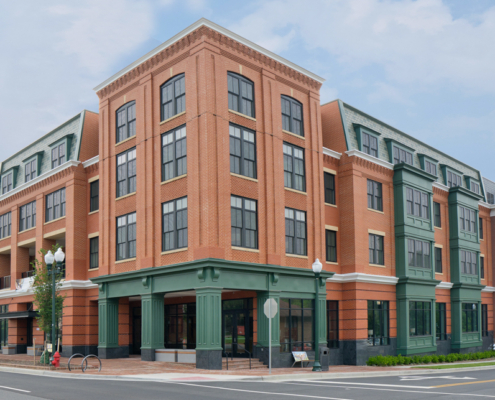The image features a large, four-story building with a classical architectural design, situated prominently at the corner of an intersection. The building's façade is a harmonious blend of orange and green: the upper levels are composed of predominantly orange brick with elegant white trim outlining the windows, while the lower level is highlighted by green paneling with large glass windows. 

The pristine street in front of the building is newly paved and marked with freshly painted lines, complementing the clean, well-maintained sidewalk made of brick. At the corner, a small flight of three to four stairs leads up to the building's entrance, which is flanked by a pair of stately street lamps. One of these lamps has a bicycle parked beside it, though no other vehicles or pedestrians are present, adding to the serene atmosphere.

Additional details enrich the setting: a fire hydrant and a stop sign are visible near one side of the corner, while shrubs and trees adorn the sides of the building, providing a touch of greenery. The structure, with its well-defined windows and doors on both visible sides, contrasts with the empty surroundings, making it almost resemble a meticulously crafted 3D model in its clarity and detail. The overall scene exudes a sense of order and tranquility, anchored by the classical beauty of the building at its center.